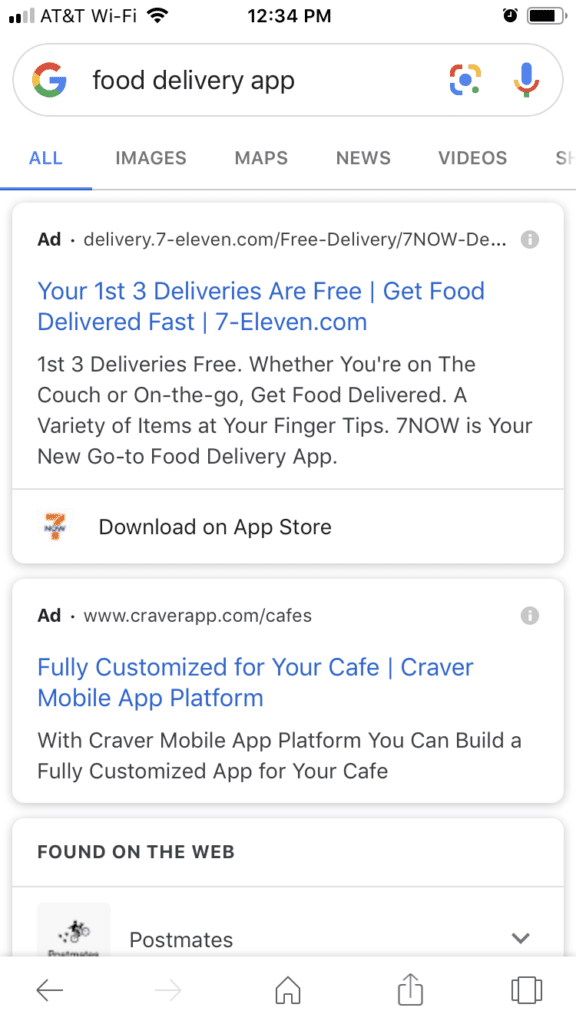This detailed caption provides a vivid description of the screenshot, ensuring all relevant aspects are thoroughly covered.

---

This screenshot, captured on an iPhone, displays a Google search results page. In the top left corner, the status bar indicates the user is on the AT&T network with two bars of cellular coverage and is connected to Wi-Fi. The time shown is 12:34 p.m., with an alarm set and approximately 80% battery remaining.

The user has searched for "food delivery app" on Google, with the search set to "All" results. Other search categories like Images, Maps, News, and Videos are visible but not selected. The primary focus of the screenshot is on the two prominent ads at the top of the search results.

The first ad is for 7-Eleven delivery service. The ad headline reads, "7-Eleven Delivery: Your First Three Deliveries Are Free." The ad text highlights the convenience of getting food delivered quickly from 7-Eleven, emphasizing, "Whether you're on the couch or on the go, get food delivered. A variety of items at your fingertips. 7-Now is your new go-to food delivery app."

The second ad is for the Craver app, with the headline, "CraverApp.com/Cafes: Fully Customized for Your Cafe." The ad promotes the Craver mobile app platform, stating, "With Craver mobile app platform you can build a fully customized app for your cafe."

Below these ads, there's a section labeled "Found on the web," where 'Postmates' appears as a search result, though the detailed description of Postmates is not fully visible in the screenshot.